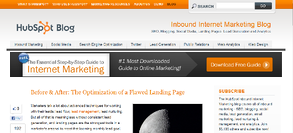This image features the HubSpot Blog website. On the top left corner, the title "HubSpot Blog" is prominently displayed. To the right of this title, the text "An Orange Inbound Internet Marketing Blog" is written. Directly below this header, a list of key topics is outlined, including "SEO," "Blogging," "Social Media," "Landing Pages," "Lead Generation," and "Analytics."

Further down the page, categories are neatly listed on the same line: "Inbound Marketing," "Social Media," "Search Engine Optimization," "Twitter," "Lead Generation," "Public Relations," "Web Analytics," and "Web Design." 

Towards the bottom is a blackish gray rectangular banner with the text "The Essential Step-by-Step Guide to Internet Marketing." The words "Internet Marketing" are highlighted in orange, while "The Essential Step-by-Step Guide to" is in a blackish gray color. Additionally, the banner includes the note, "The Number One Most Downloaded Guide to Online Marketing."